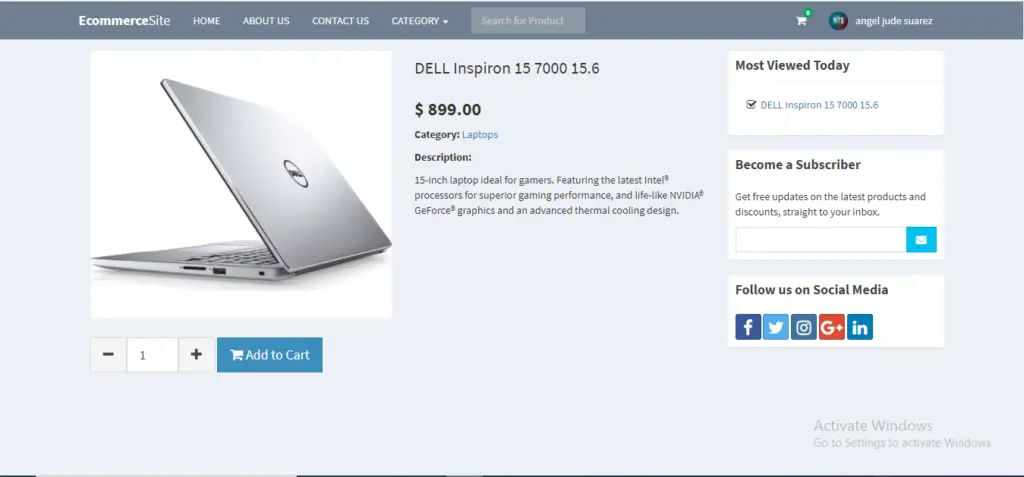On an e-commerce website, a detailed product page showcases a Dell Inspiron 157000, a 15.6-inch laptop listed at a sale price of $899. The top navigation bar includes links to 'Home', 'About Us', 'Contact Us', 'Category', and a search bar labeled 'Search for Product'. The user currently logged in is Angel Jude Suarez.

The laptop, categorized under 'Laptops', is a sleek gray model with specifications designed to attract gamers. It boasts the latest Intel processors, NVIDIA GeForce graphics for lifelike visuals, and an advanced thermal cooling design to ensure optimal performance during intense gaming sessions. Customers can adjust the quantity and add the laptop to their cart directly from this page.

To the right of the product description, a section indicates that this item is the 'Most Viewed Today'. Below this, there's an invitation to become a subscriber, offering free updates on the latest products and discounts delivered straight to one's inbox. The page also encourages users to follow the store on various social media platforms, including Facebook, Twitter, Instagram, Google, and LinkedIn, with corresponding icons provided.